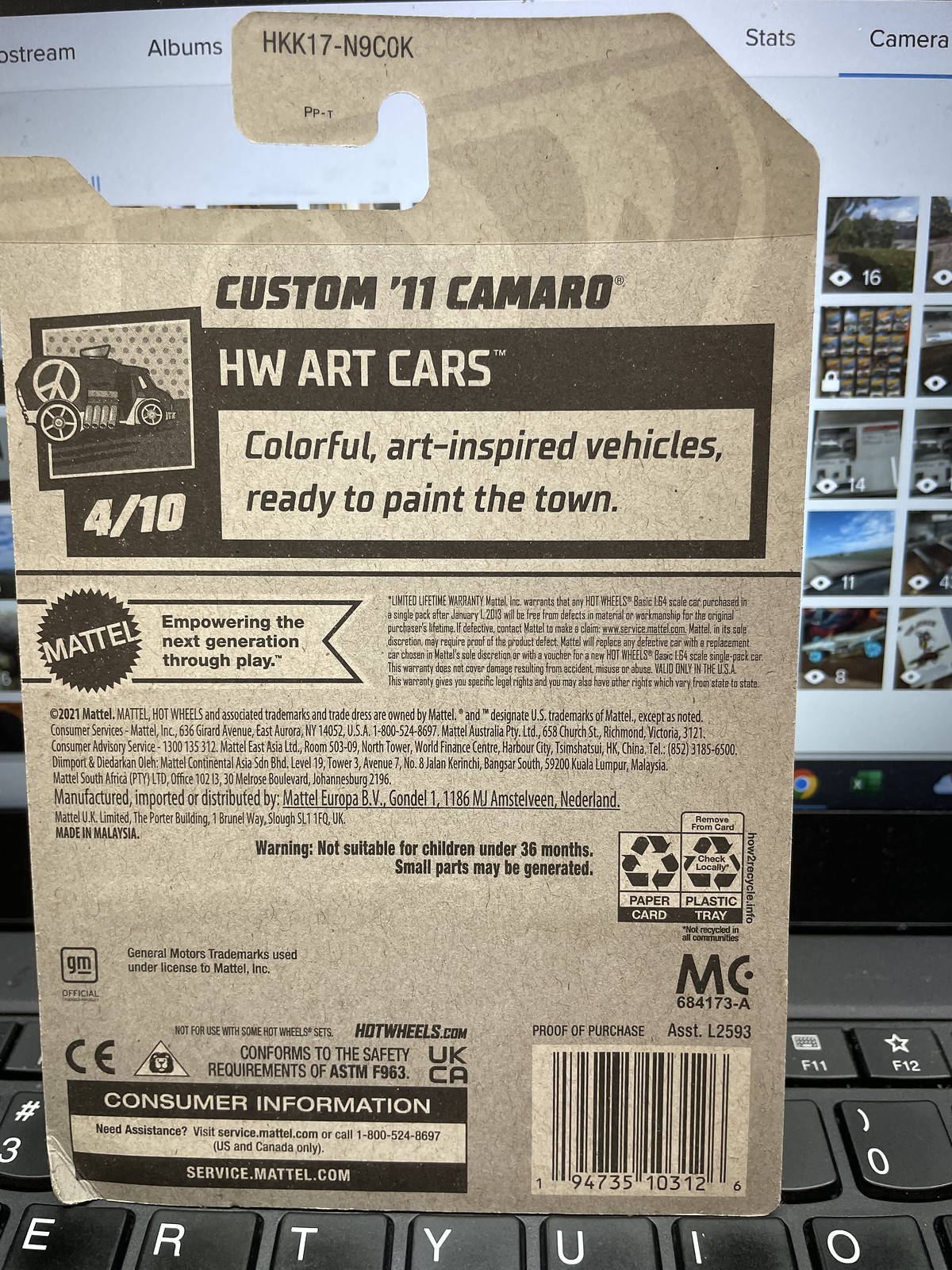In this image, the primary focus is the back packaging of a product, identified as a Custom '11 Camaro from the HW Art Cars series by Mattel. The packaging highlights "Colorful Art Inspired Vehicles, Ready to Paint the Town," emphasizing the creative and playful nature of the toy. Positioned centrally in the image, this product is surrounded by various colors including black, white, gray, blue, yellow, orange, and light blue. A small, unreadable text is present, along with a 4-10 rating, likely indicating a categorization of the product. At the bottom right corner, a barcode is visible for scanning purposes. The background of the image features an open laptop displaying a black keyboard and several indistinct images on its screen, suggesting an indoor setting, possibly a computer room. The caption also notes Mattel's tagline, "Empowering the next generation through play," reinforcing the brand's mission.